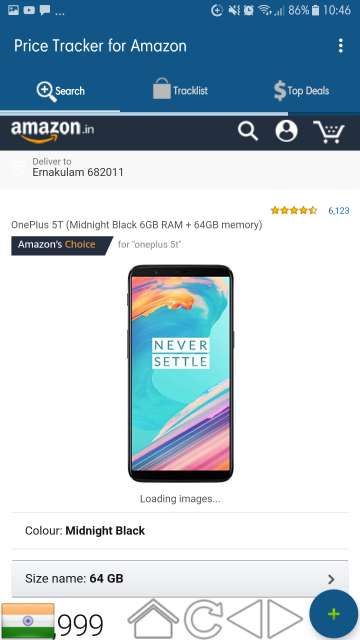Displayed on a mobile phone screen is an Amazon webpage, notable for its detailed layout and rich visual elements. At the very top of the screen, within a thick blue band, several icons are aligned in the left corner, including the YouTube, text, and photo applications. Towards the right, beginning around the middle of the top bar, there are a series of icons: a plus sign within a circle, a no sound indicator, an alarm icon, a Wi-Fi signal, signal bars, a battery display showing 86%, and the current time, 10:46. Below this section, a title reads "Price Tracker for Amazon" accompanied by a vertical menu with three stacked dots on the right side.

Further down, the navigation bar includes options for navigating, searching, accessing the track list, and viewing top deals, with the search function likely being active. Underneath this, a black strip prominently displays "Amazon.in" along with options for the search profile and cart. The shipping address is specified as "Deliver to EMAKULAM 682011."

The product details follow: "OnePlus 5T," described as having a Midnight Black finish, 6GB of RAM, and 64GB of memory. It boasts an impressive rating of five and a half stars from 6,123 reviews and is marked as an Amazon Choice for OnePlus 5T. The product image shows a sleek smartphone with the slogan "Never Settle" on its screen, which features an abstract background composed of vibrant turquoise, orange, and pink hues.